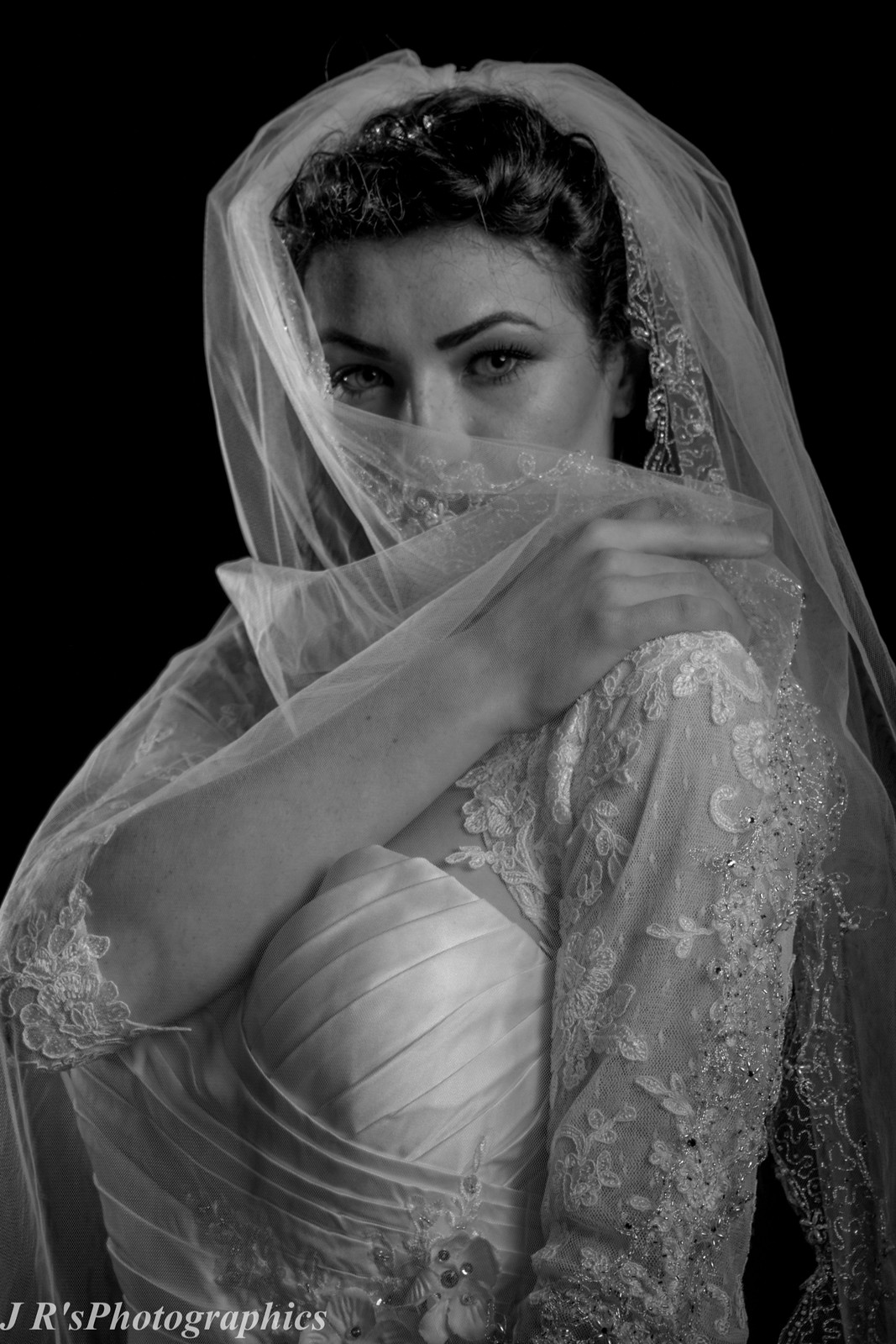This black-and-white image showcases a striking bridal portrait with a solid black background that emphasizes the bride at the center. The scene is lit dramatically, focusing on the details of the bride's attire. She wears an elegant wedding dress with three-quarter length, see-through sleeves adorned with intricate designs. The dress features delicate stripes and floral embellishments. The bride has dark hair and light-colored skin, and her eyes gaze directly into the camera, creating an intimate connection with the viewer. She partially covers her face with the veil, which drapes from the back of her head across the front of her face, adding an air of mystery. The bride's bare hands are visible at the forearm level, one of which holds the veil in place. At the bottom left corner of the image, the text "JR's Photographics" credits the photographer. This professional photoshoot captures the timeless elegance and intricate details of a Christian bridal dress against a contrasted black backdrop.